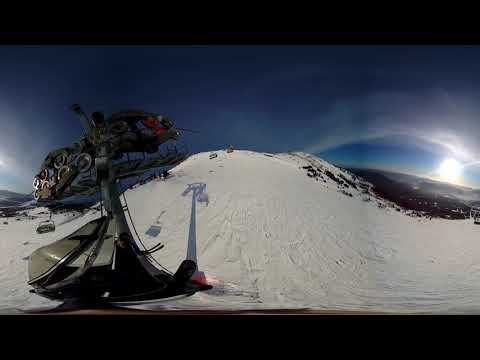The image captures a snowy, mountainous landscape, taken from the perspective of someone riding a ski lift. The scene is bathed in bright natural light under a clear blue sky, with the sun setting in the background, casting a deep silhouette and long shadows. The foreground features a sloping snow-covered hill, marked by ski trails. On the left side, there's a complex, insect-like metallic mechanism attached to the ski lift tower, in motion, partly obscured by the extreme fisheye lens distortion. Above, the ski lift chair and cables can be observed, emphasizing the lift's height. The overall atmosphere is serene yet dynamic, with the stark white of the snow contrasting against the blue sky and metallic elements.